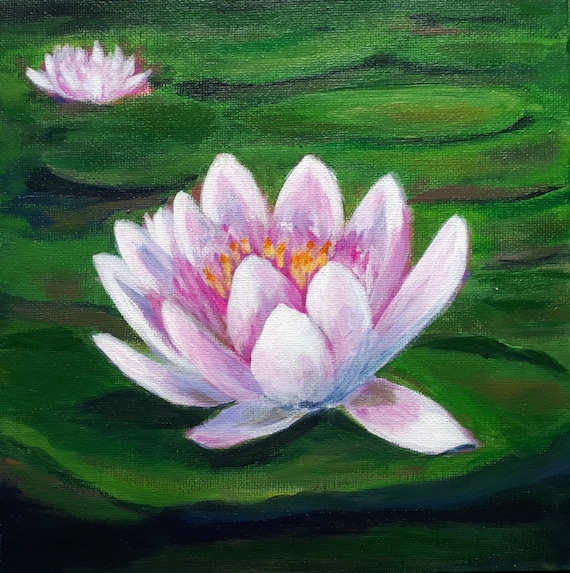The image is a detailed painting of water lilies in a lily pond. At the center is a prominent pink water lily with approximately 12 delicate petals, each with hints of orange and white shading, and faint touches of purple. It rests on a dark green or forest green lily pad that occupies a significant portion of the bottom half of the image. Surrounding this central scene are numerous green lily pads floating on the water’s surface, with about six or seven partially visible pads in the upper section of the painting. In the top left corner, there is a smaller pink water lily, also resting on a green pad. Overall, the composition is filled with these large green pads extending across the water and two distinct pink water lilies, highlighting the serene beauty of this aquatic scene.